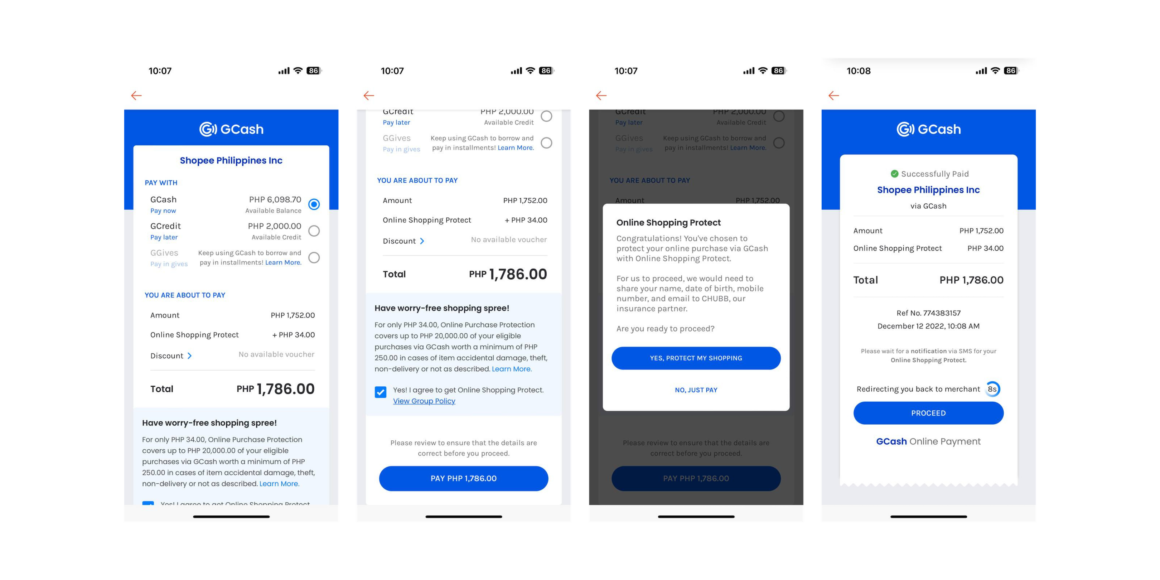This series of small screenshots showcases various features of the GCash app, a popular mobile wallet service in the Philippines. The images contain an abundance of textual information, predominantly in Filipino currency (PHP). The first few images include mostly white backgrounds accented with blue buttons and blue-themed elements along the edges. These screenshots appear to focus on money-transfer or currency conversion functionalities within the app. 

In the third screenshot, a pop-up window is visible with the headings "online shopping" and "protect." The pop-up provides an option to either safeguard the user's shopping experience with a "Yes, protect my shopping" button or a "No, not now" button. 

The last screenshot displays a summary screen, indicating a total amount of PHP 1,786, with a "Proceed" button at the end, suggesting the finalization of a transaction. The exact value of PHP 1,786 in dollars is not clear from the screenshots. Overall, the images illustrate a dense and detailed interface designed to facilitate various financial transactions through the GCash app.